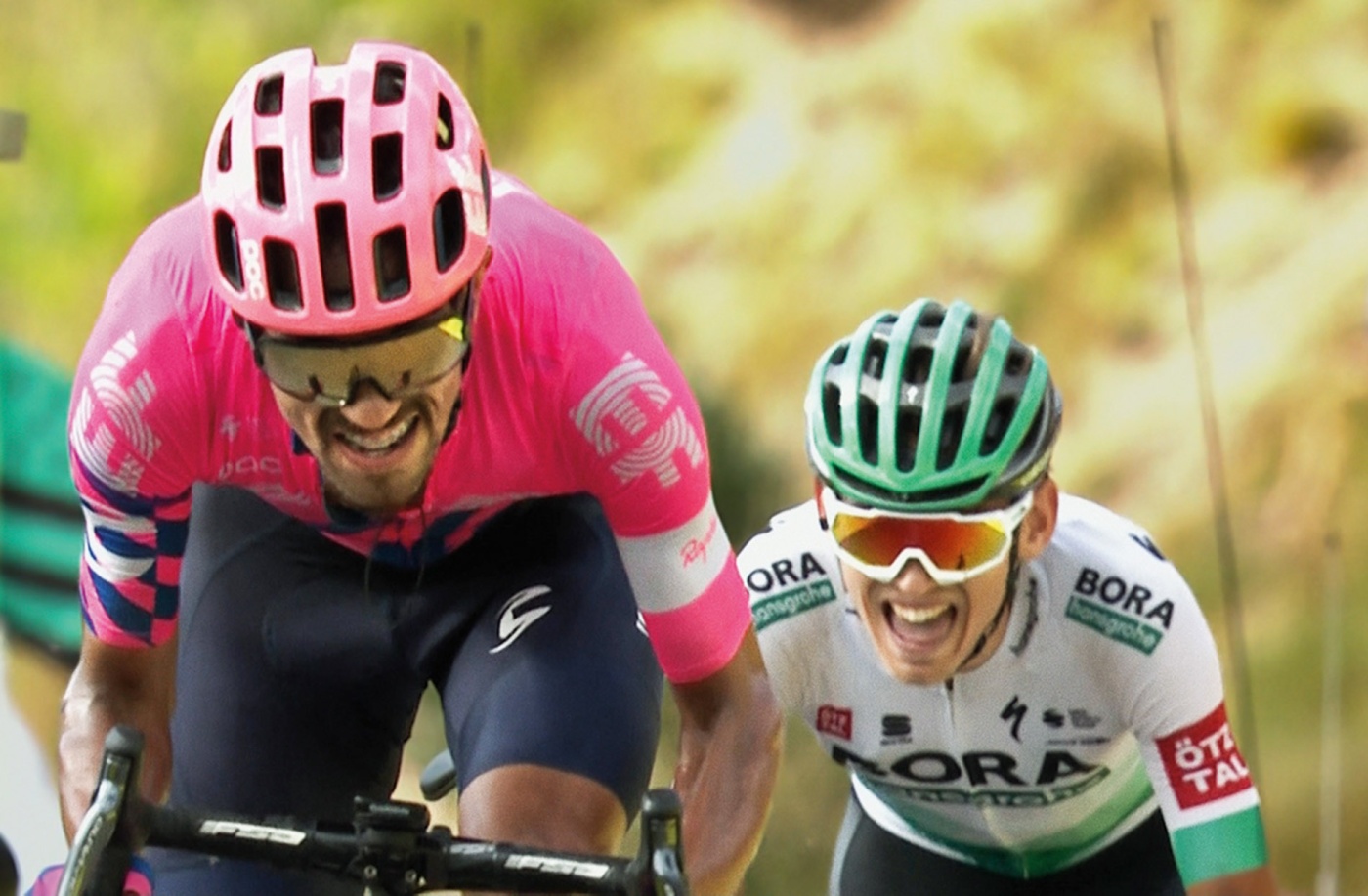In this vivid outdoor photograph, we see two cyclists competing intensely on a bright, sunny day, captured from a front-facing angle. The blurred green foliage in the background, with sunlight filtering through the leaves, emphasizes the speed and focus of the riders.

The primary rider on the left wears a pink and black helmet paired with reflective black sunglasses. His outfit consists of a pink jersey with white lettering "EF" on both sleeves, and black racing shorts. He's hunched over his black handlebars, gripping each side firmly with one hand, his mouth slightly open, indicative of his exertion.

To his right, partially behind him, is another cyclist, sporting a mint-green and black helmet. He wears distinctive white visor glasses with yellow-orange lenses, complementing his white jersey adorned with mint-green accents and a red, square logo, along with black shorts. This rider too is hunched over his handlebars, his mouth open in a mix of a smile and effort as they both race forward.